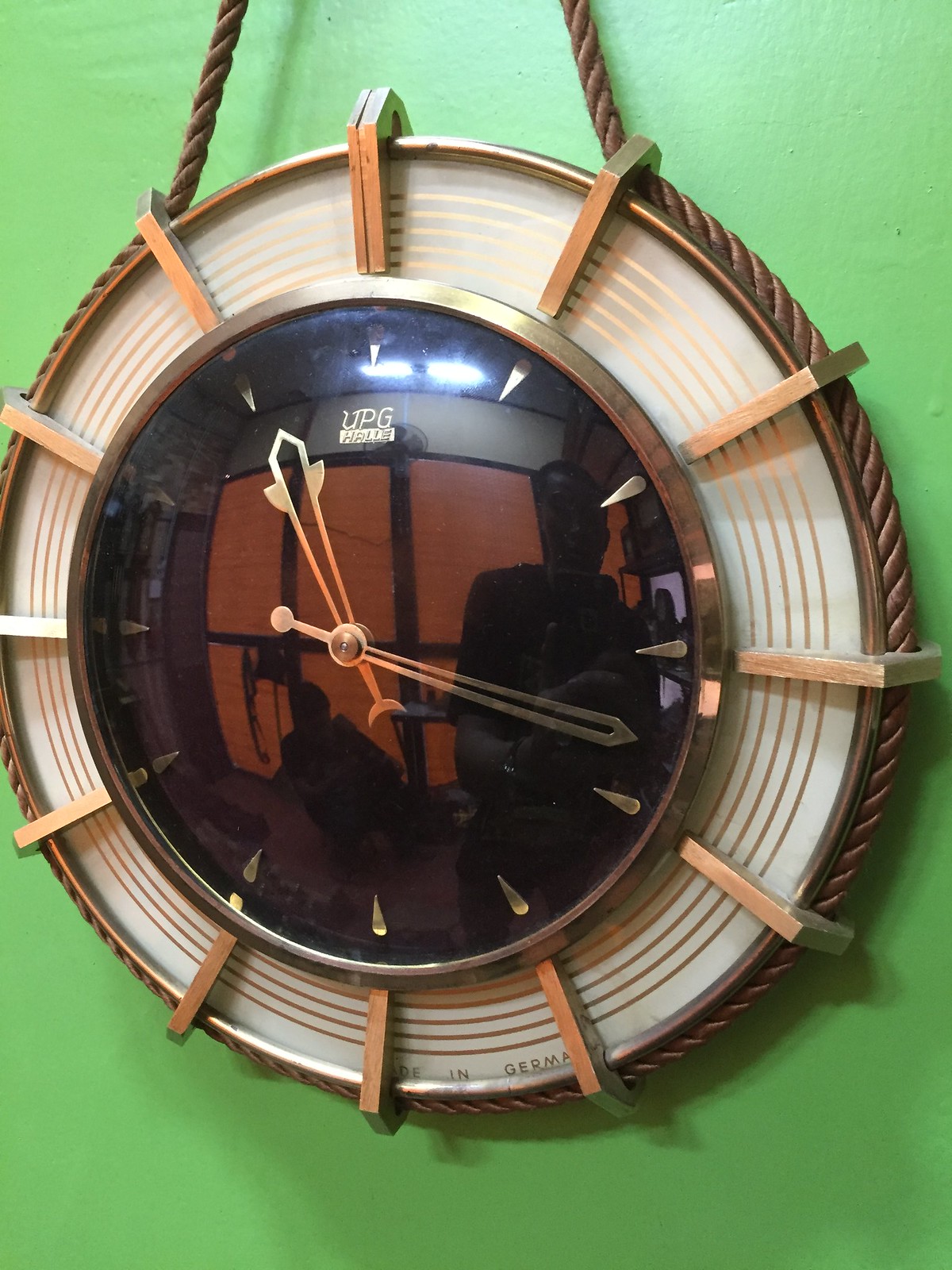A unique clock designed with a rope encircling its circumference. The rope threads through the hour markers, which resemble elongated, bronze-colored metal hooks. Engraved near the bottom edge of the clock's face is the inscription "Made in Germany." Surrounding the bezel are five concentric gold circles, complementing the brass-bronze hue of the overall design. The clock's face and structure seem conical or spherical in shape. The hour and minute hands feature intricate open grooves and shapes, matching the bronzy, brassy color scheme. Adjacent to the hour holders on the bezel are the hour indicators. The clockmaker, identified by the inscription "UPG," showcases meticulous craftsmanship in this extraordinary timepiece.